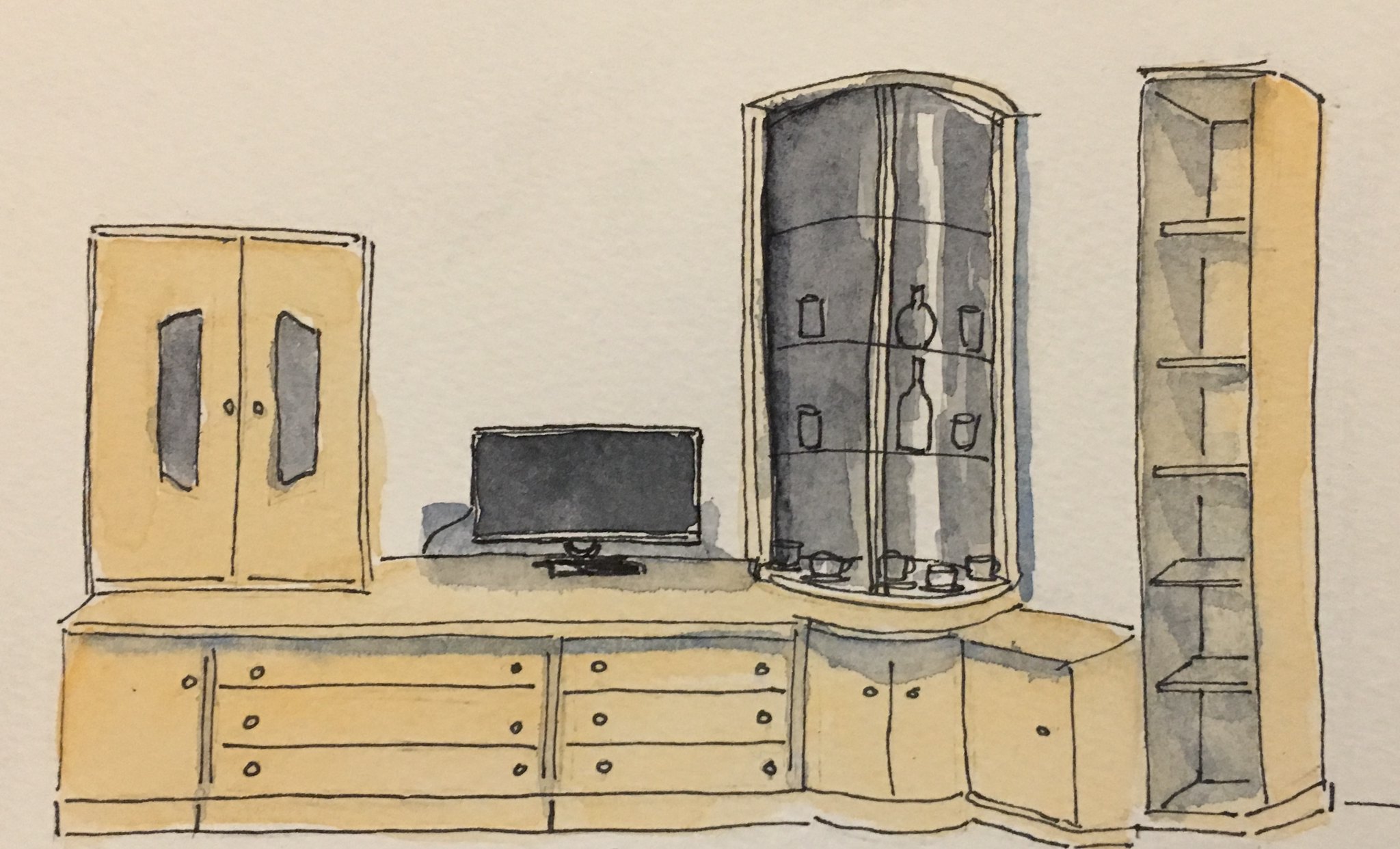This image depicts a detailed sketch of a media center or living room setup. Central to the scene is a small, flat screen TV or computer monitor positioned atop a tan or yellowish-tan desk unit. The desk itself features six horizontal drawers with small black circular knobs. To the left of the desk, there is a cabinet with double doors. On top of the desk, to the left of the TV, sits a small cabinet with two drawers and a black glass front.

To the right of the TV, there's a curio cabinet, also with black glass, revealing shelves inside. The contents of this curio cabinet include a variety of items such as glasses, teacups at the bottom, and a couple of wine bottles in the middle shelves. Further to the right of this cabinet is an empty shelving unit with six shelves, matching the tan or yellowish theme of the entire unit. The scene is set against a light-colored wall, casting shadows that enhance the depth and details of the sketch. The overall style is cartoonish or animated, adding a whimsical touch to the detailed representation.